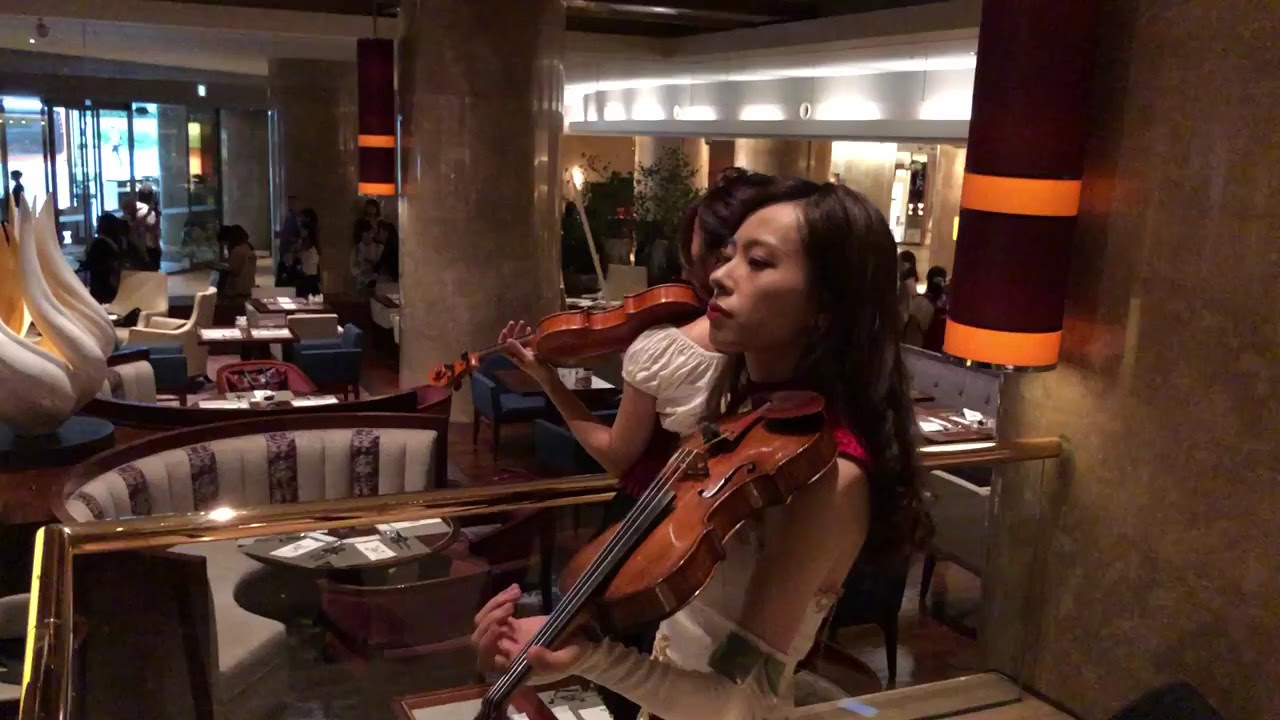The color photograph, presented in a landscape orientation, showcases an interior view of a modern restaurant or cocktail lounge. In the center foreground, a young woman with long dark hair and dark skin, wearing a white blouse, plays a wooden violin propped on her shoulder. Beside her, slightly back, another similarly dressed woman with dark hair and an Asian appearance also plays a violin, facing away from the camera. Both appear engaged in their music. The women are near a glass partition with a gold banister, separating them from the lower section of the restaurant.

The background reveals a modern setting with polished stone pillars and semi-circular banquette-style tables adorned with gray cushions and black stripes. Orange bands on sconces mounted to the large marble-textured columns add a splash of color. A purple and orange light also accentuates the contemporary vibe. The restaurant isn't particularly crowded, but a few patrons are visible, along with some people reflected in a distant mirror. The space to the right, partially visible, features bright lighting and several plants, while the top left background shows large glass doors leading outside. The detailed design elements contribute to an overall ambiance of polished sophistication and realism.